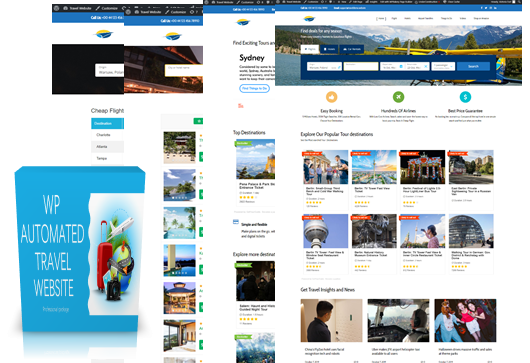The image depicts a VIP automated travel website with a clean, white background. Several webpages or tabs from the site are overlaid, creating a slightly cluttered appearance. Prominently displayed on one of the top pages is a destination focus on Sydney. The website offers various vacation packages, including destination options and flight booking choices. User reviews with star ratings are visible, indicating a system for gauging customer satisfaction. The pages also showcase images of locations and events available for booking as part of travel packages. In the bottom left corner is the website's logo, featuring a medium blue color and an airplane icon. Despite the overlapping pages making some details difficult to read, the overall impression is of a comprehensive and user-centered travel booking platform with multiple vacation options and amenities.